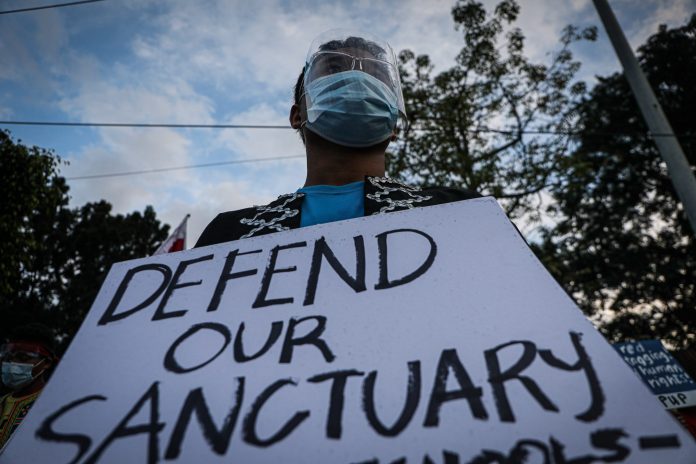This color photograph captures a male protester holding a white cardboard sign with the partially obscured message "Defend Our Sanctuary" written in black marker. The unique low-angle shot, taken from waist level, looks directly up at the man, emphasizing the protest's atmosphere. He's equipped with comprehensive COVID-19 protective gear: a blue mask, glasses, and a clear face shield. He has short dark hair and wears a blue shirt beneath a black sweater adorned with white decorations. The backdrop includes a blue sky with diffused, fluffy clouds, various trees, and a telephone pole with exposed wires. Another potential protest participant is partially visible in the right foreground, holding a sign. The lighting suggests either midday or the onset of sunset.